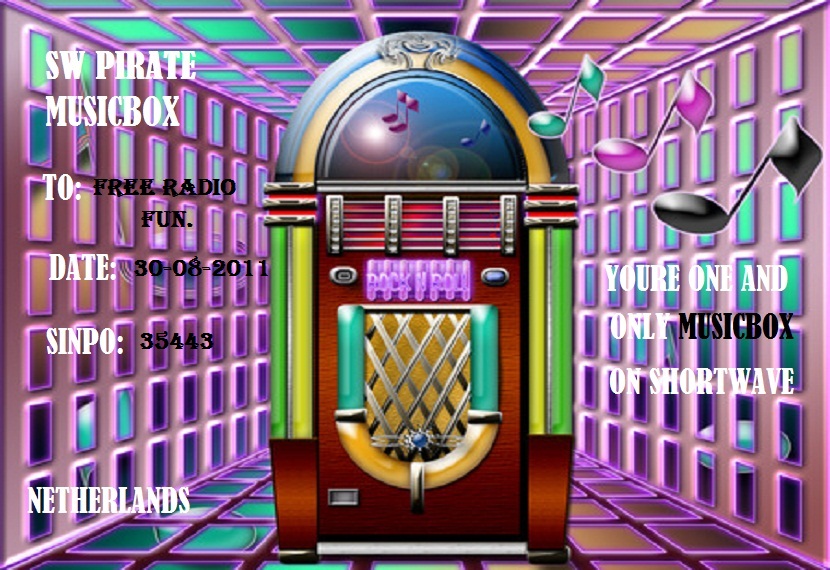This poster presents a striking, digitally rendered image featuring a colorful jukebox at its center, set against a vibrant backdrop. The jukebox itself is an eye-catching piece with a semicircular, blue and gold dome and sides painted in green and light yellowish hues, while the main body is fashioned from redwood adorned with a silver grill flanked by green accents and a yellow U-shaped base. Above the jukebox, a smattering of purple, green, pink, and black musical notes adds to the lively composition. The background is characterized by a pink, metallic net-like pattern that encloses the central structure and extends to the sides, top, and bottom, amplifying the sense of a three-dimensional space.

Text is strategically placed on both sides of the image. On the left, the text reads:
"SW Pirate Music Box 2
Free Radio Fun
Date: 30-08-2011
SINPO: 35443
Netherlands"

On the right side, the text promotes the central theme with:
"Your one and only music box on shortwave."

The overall aesthetic suggests an advertisement for a radio station, leveraging the vibrant digital artistry to draw attention and convey a sense of fun and entertainment. The color palette is diverse, showcasing shades of purple, pink, green, blue, black, white, grey, yellow, tan, and brown. The rectangular format of the poster, being slightly wider than tall, further enhances its visual impact, drawing the viewer into its colorful, musical world.